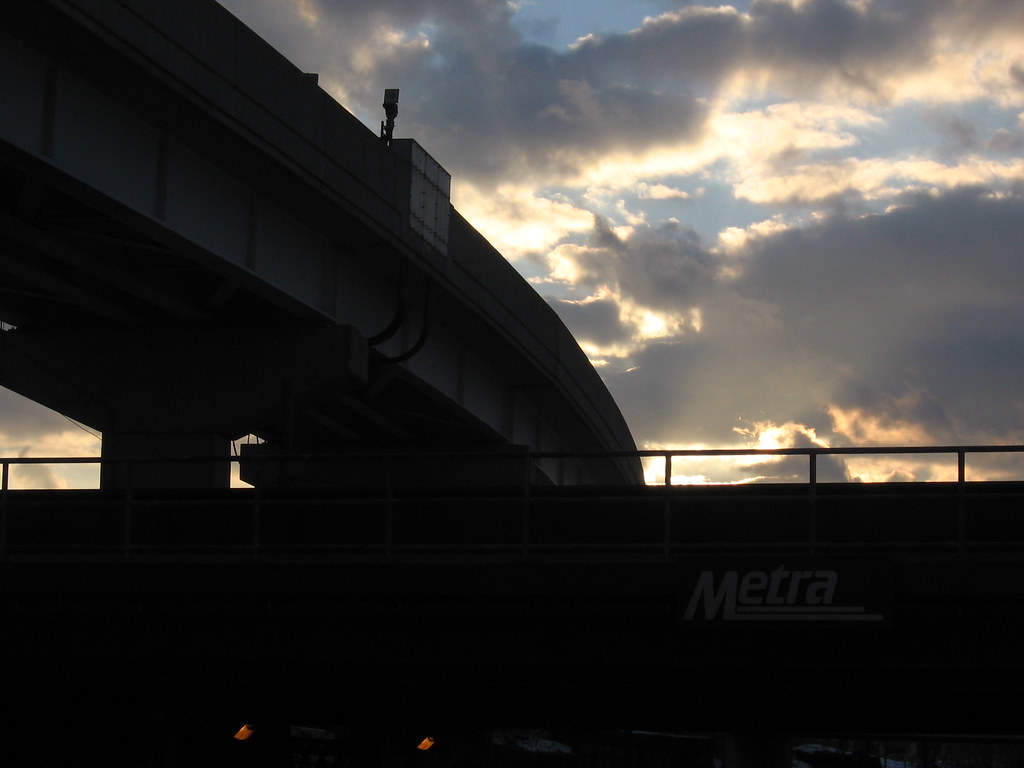The photograph captures a striking outdoor scene during sunset, where a cloudy skyline dominates most of the composition. The gray clouds, tinged with bits of light from the setting sun, create a contrasting backdrop against the dark, almost black, elements below. This area of the image features indistinct black silhouettes that suggest industrial structures, including an overpass or a bridge, with possible concrete columns and metal bars jutting out. The structure appears complex, with parts of it appearing to wrap from the top left corner down towards the middle. The rest of the image below the skyline is enveloped in deep shadow, making specific features difficult to distinguish. In the bottom right-hand corner, a white label that reads "METRA" with two underlines is visible, while the bottom left-hand corner features two small orange dots, adding subtle splashes of color to the otherwise monochromatic scene. The image's rectangular dimensions are slightly wider than tall, framing this dramatic contrast of light and dark.